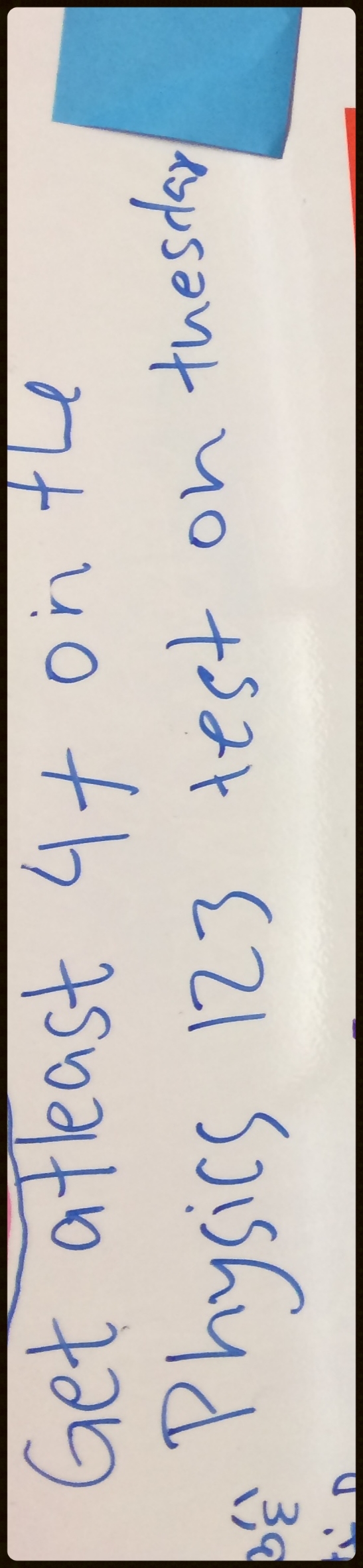The photograph depicts a whiteboard with various notations written in blue marker. Predominantly, the words "GET at least four plus on the PHYSICS one two three test on Tuesday" are inscribed, with "GET" and "PHYSICS" emphasized in capital letters. However, the word "Tuesday" lacks capitalization and appears compressed towards the end, likely due to the presence of a dark blue post-it note positioned at the far right edge of the board.

In the bottom left corner, there are additional markings that seem to represent a "B" and possibly an "E," accompanied by several diagonal lines that might indicate a chemical formula. Below these characters, two dots and a small vertical line create a simple, face-like design. 

The image captures a slight reflection of fluorescent lights at the very bottom, suggesting the setting is a classroom with similar lighting fixtures on the ceiling.